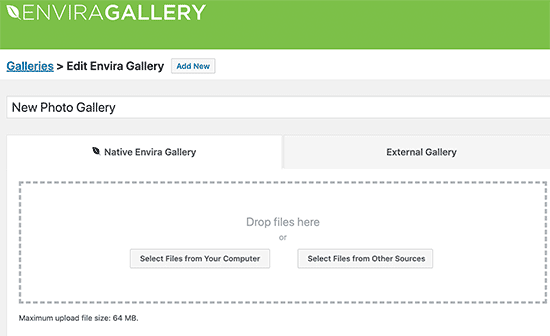This image is a detailed screenshot of a webpage belonging to "Envira Gallery," a platform for uploading and managing photos in a personal gallery. The top section of the page features a green header, prominently displaying the site's name. Below the header, the page has a clean white background. 

At the center of the page, a large rectangular drop zone is present, designed for users to drag and drop files for upload. Additionally, there are two alternative options for uploading files: one for selecting files directly from the user's computer, and another for choosing files from other sources. In the bottom left-hand corner of the page, there is an important note stating that the maximum upload file size is limited to 64 megabytes. The overall layout is intuitive, providing a straightforward user experience for those looking to add images to their personal galleries on Envira Gallery.